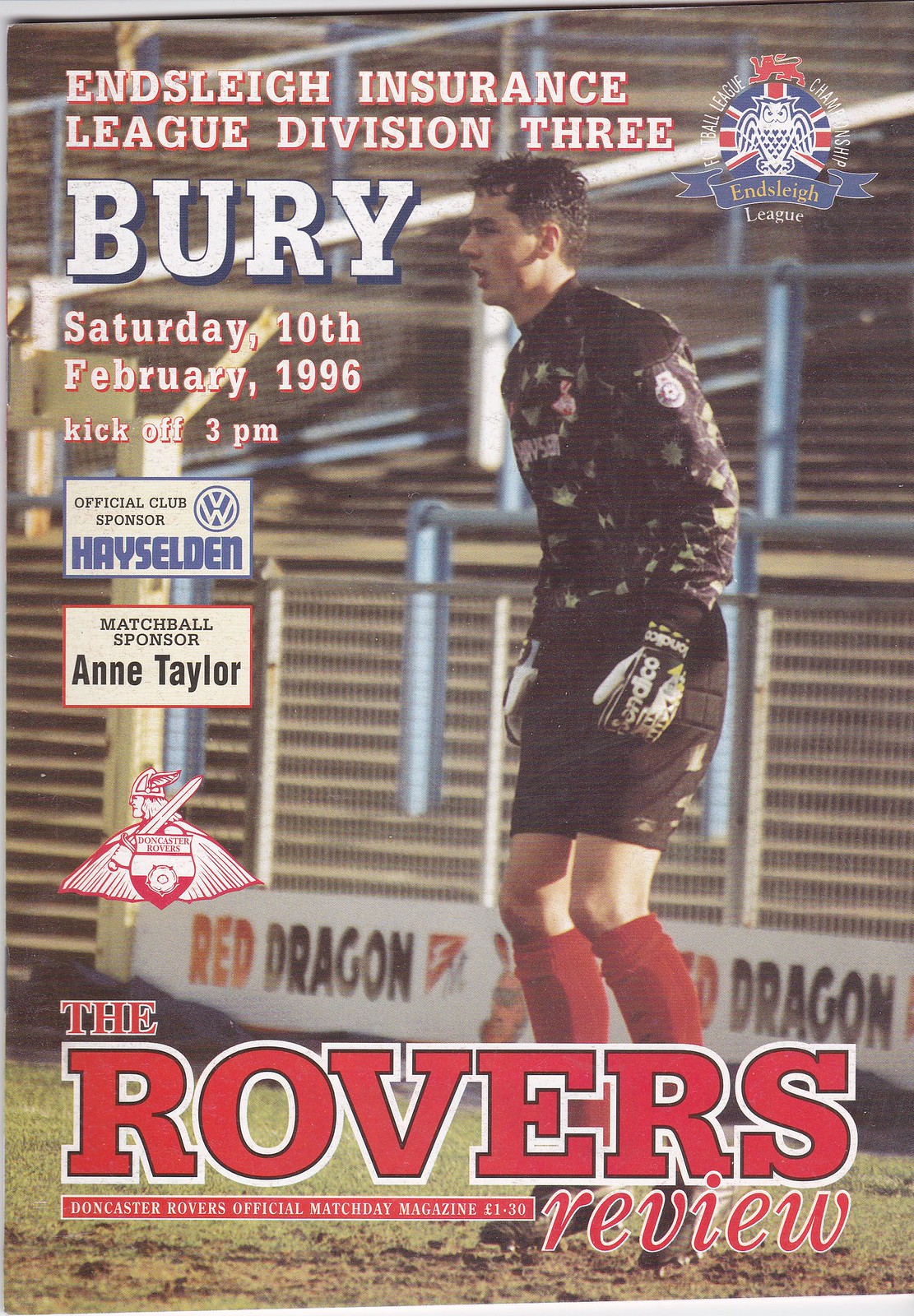The image depicts the front cover of a soccer program known as "The Rover's Review." The program features a photograph of a soccer player, likely a goalie given his gloves, standing on a soccer field, with the backdrop of stadium stands. The man is captured mostly in profile, his gaze directed off to the side. He is a white male with short, dark hair, dressed in a black outfit with greenish accents on the upper part of his shirt. His shorts are black, he is wearing red socks, and he has black and white gloves.

Text on the program indicates it is for a match in the Ainsley Insurance League Division III, between Doncaster Rovers and Bury, scheduled for Saturday, 10th February 1996, with kickoff at 3:00 p.m. The cover also features various sponsor advertisements, including the Official Club Sponsor VW and Match Ball Sponsor Ann Taylor. The Doncaster Rovers club logo, which portrays a Viking holding a sword and wearing a helmet with wings atop a shield, is prominently displayed. Additionally, the program is priced at £1.30 and includes mention of the Football League Champions Enslay League, signified by a logo featuring an owl and a lion.